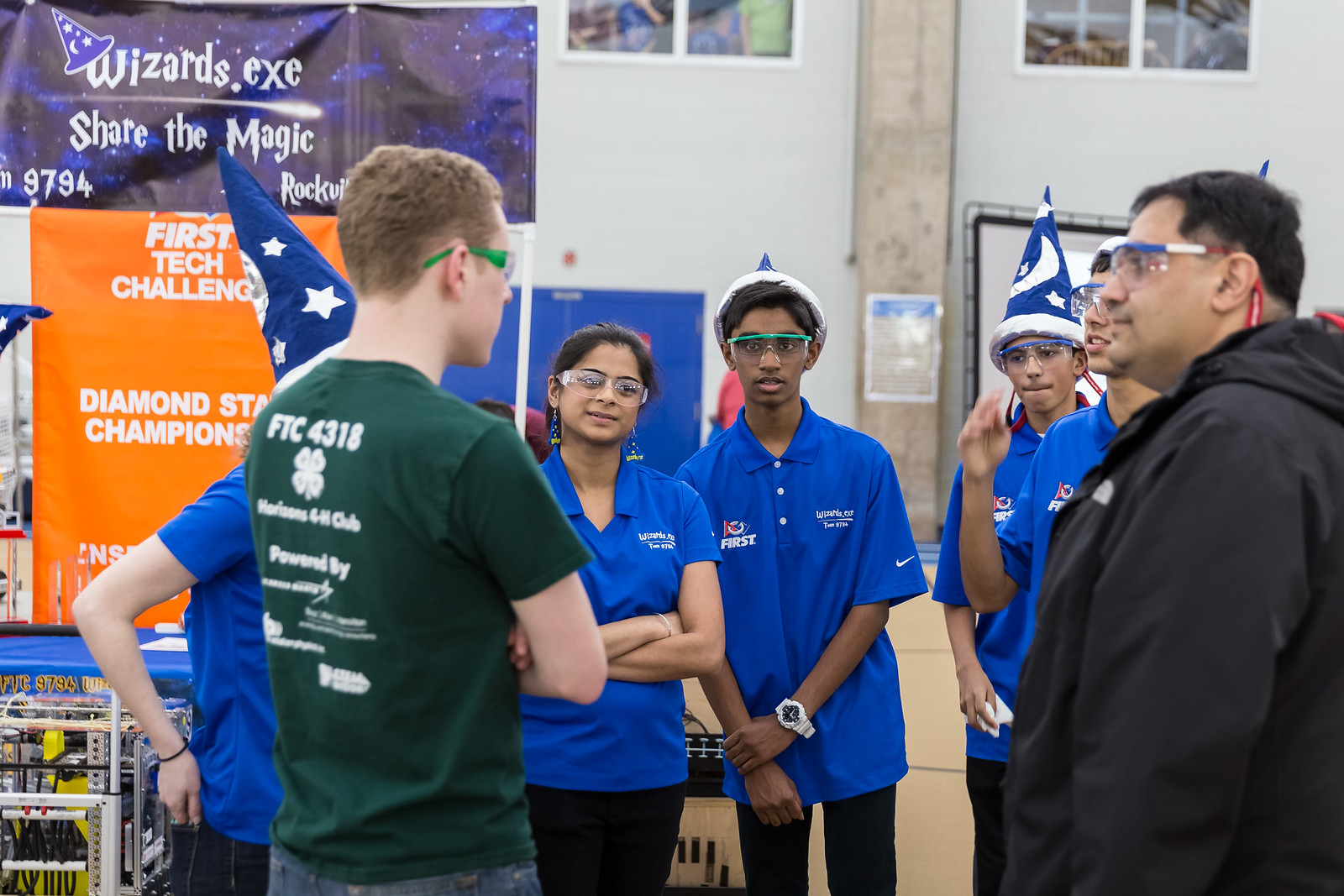In the image, there is a diverse group of young people gathered in a semi-circle, possibly engaged in a meeting or discussion. Most of the group members are wearing matching blue button-up shirts and pointed wizard hats adorned with stars and moon crests, reminiscent of Mickey Mouse's wizard hat in Fantasia. These uniforms bear logos with text that says "Wizards.exe, Share the Magic" and "FIRST", indicating they are part of the FIRST Tech Challenge. 

In the top left corner, there is a dark blue and black banner displaying "Wizards.exe" with "Share the Magic" below it, accompanied by the number "9794". Beneath this banner, an orange vertical rectangle sign reads "FIRST Tech Challenge, Diamond State Champions". The background features white walls and a blue table, accentuating a typical event setting.

Among the group, a boy in a green shirt stands out; his shirt features the text “FTC 4318” with a four-leaf clover and some unreadable smaller text. Another older man in a black hoodie and safety goggles, possibly a mentor or teacher, is also present. This setting depicts a tech or robotics competition with a whimsical, wizard-themed twist.